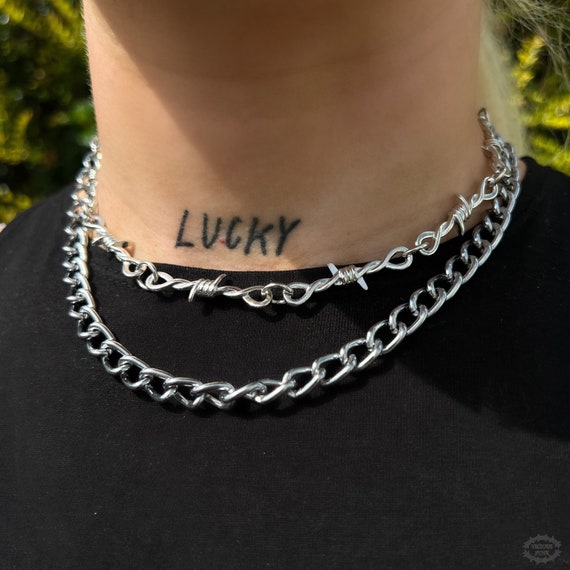This is a close-up photograph of the neck and upper chest of a Caucasian man, wearing a black shirt. The image prominently features a black tattoo on his neck that reads "LUCKY" in uneven, amateurish block letters. The tattoo appears to be written across a scar. Around his neck, the man wears two silver necklaces; the top one is designed to resemble barbed wire, while the lower one is a chain link. In the background, there is a hint of blonde hair, possibly a ponytail, and some indistinct greenery in shades of dark, light, and shadowy green, suggesting an outdoor setting with trees or pine limbs.